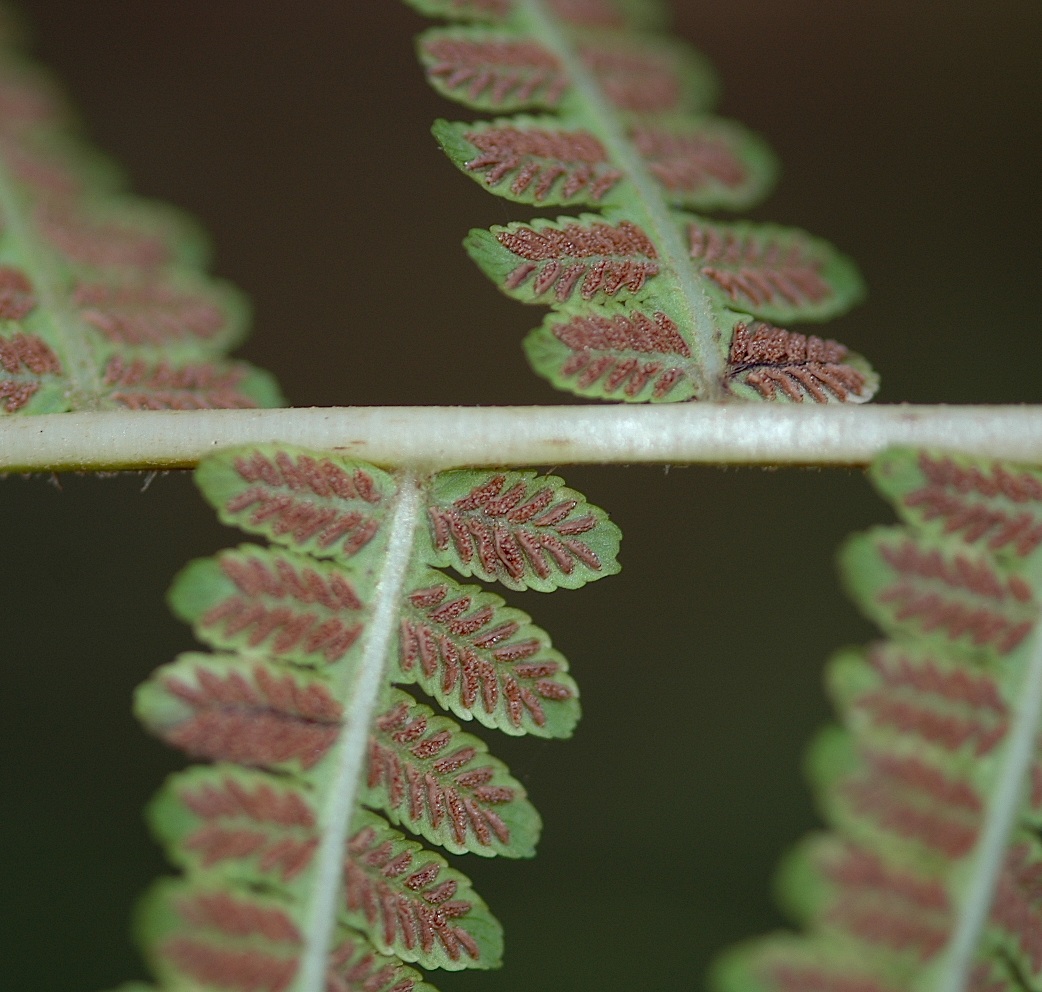This highly detailed, color photograph in a square format captures an extreme close-up of a central fern frond of what appears to be an Ancestia species. The central stem, a light beige-green hue, stretches horizontally across the middle of the image. From this stem, four partially visible branches fork out: two upward and two downward. Each branch carries intricate, medium-green fern leaves bedecked with rows of dark brown, fuzzy, spore-like patches that reflect the compound nature of ferns. The leaves centrally focus on a vivid, textural play between the green foliage and the brown spore patterns, creating a blurred, gradient effect towards the edges of the image. The background sets a deep green tone, enhancing the sharpness and realism of the ferns, suggesting the photographic style is representational realism.